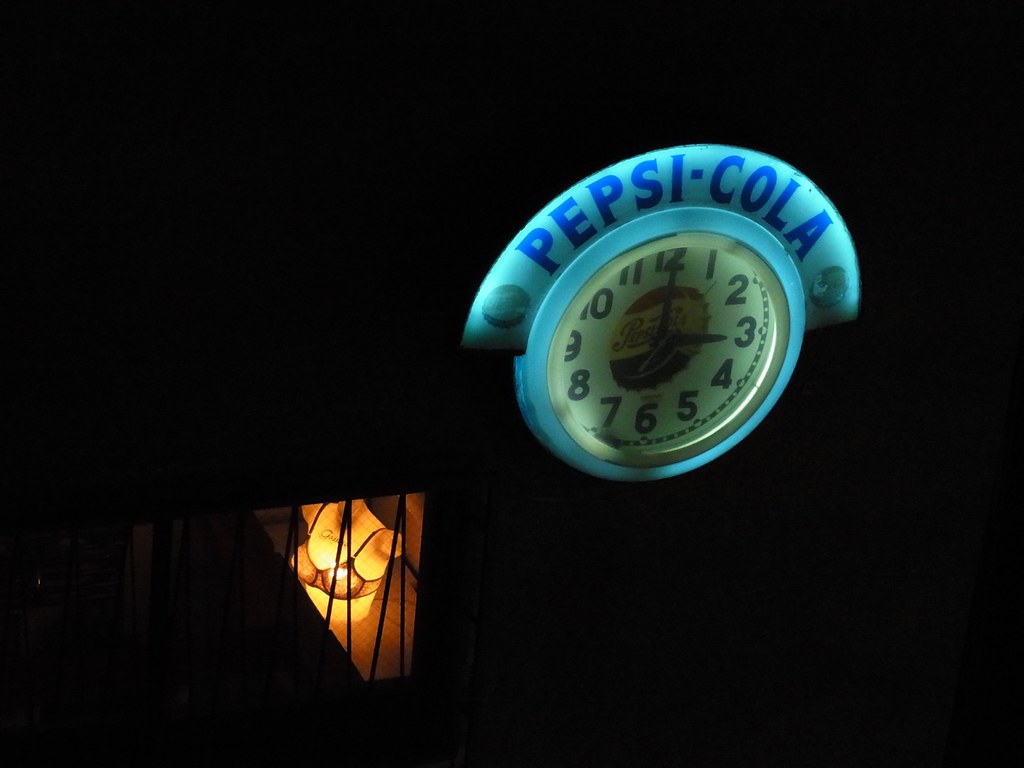The image depicts a vividly illuminated clock sign against a pitch-black background, resembling a night scene. The circular clock is outlined with a blue light, with a white face on which dark blue numerals are displayed in a standard 1 through 12 sequence, indicating a time of approximately 3 o'clock. Dominating the clock's center is an old-fashioned Pepsi-Cola bottle cap graphic, featuring the iconic red, white, and blue colors. Above the clock's face, the text "Pepsi Cola" is prominently displayed in blue, flanked by images of bottle caps. To the left of the clock, a window reveals an interior space partially lit by a yellowish light, showcasing a mannequin modeling a bra. This window also casts a glow that contrasts with the otherwise entirely black surroundings.